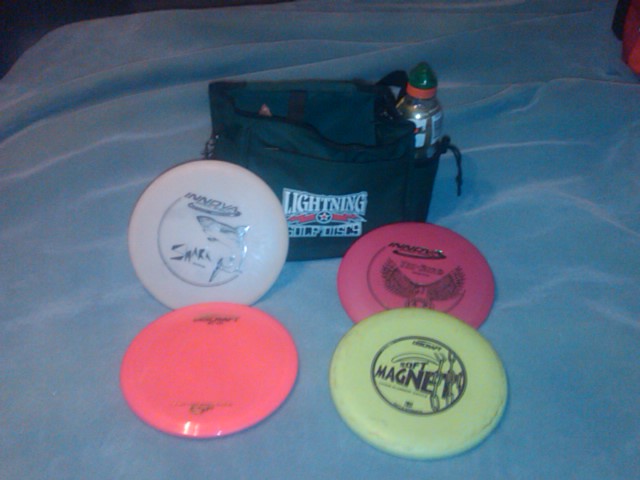In this photograph, we see a light blue blanket, possibly spread on a bed or couch, serving as the backdrop for an arrangement of disc golf essentials. Centrally positioned at the top is a green cloth tote bag marked with "Lightning Golf Disc 9," which appears to be an ample outdoor to-go bag, designed for carrying the disc golf gear. Peeking out of the side pocket of this bag is a bottle, likely a sports drink such as Gatorade.

Arrayed in front of the bag are four colorful disc golf frisbees, each displaying distinct logos and brand names. There is a white frisbee leaning against the bag, adorned with the "Shift Magnet" logo. Below it lie three more discs: an orange one, a yellow one labeled "Anaya," and a pink one. The colors bring vibrancy to the scene, highlighting each item’s unique brand and purpose. All of these details combine to portray someone gearing up for a disc golf session, with their equipment thoughtfully laid out and ready for action.